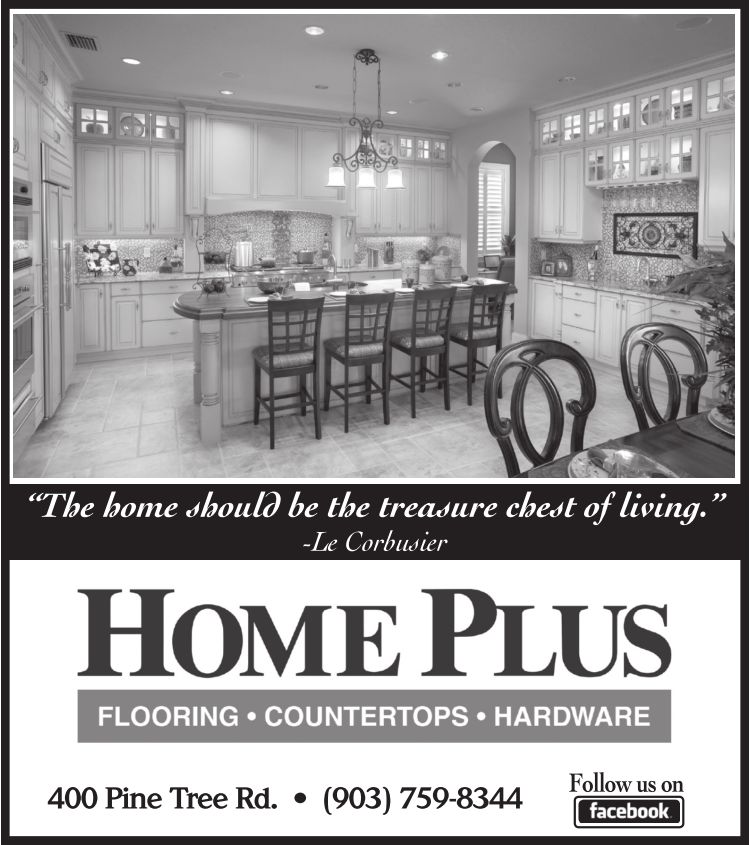The black-and-white advertisement features a photo of a brand-new, stylish kitchen occupying the top half of the image. Central to the kitchen is a breakfast bar adorned with wooden chairs, and a chandelier hanging above it. The layout includes visible cabinets and cupboards, with a double oven and an archway leading to another room on the right side. In the bottom right corner of the photo, there are two more chairs situated against a dining table. The visual portrayal of the kitchen is framed by windows that bring natural light, highlighting the contemporary interior.

Beneath the photograph, a black banner with white text features a quote by Le Corbusier: "The home should be the treasure chest of living." Below this banner, on a white background with black block capitals, the text reads "Home Plus." A grey banner with smaller white text underneath lists the services offered: "flooring, countertops, hardware." Further down, the text provides the business location and contact number: "400 Pine Tree Road, 903-759-8344." In the bottom right corner of the advertisement, a note in black text encourages viewers to "follow us on Facebook," with the word "Facebook" displayed in its iconic logo.